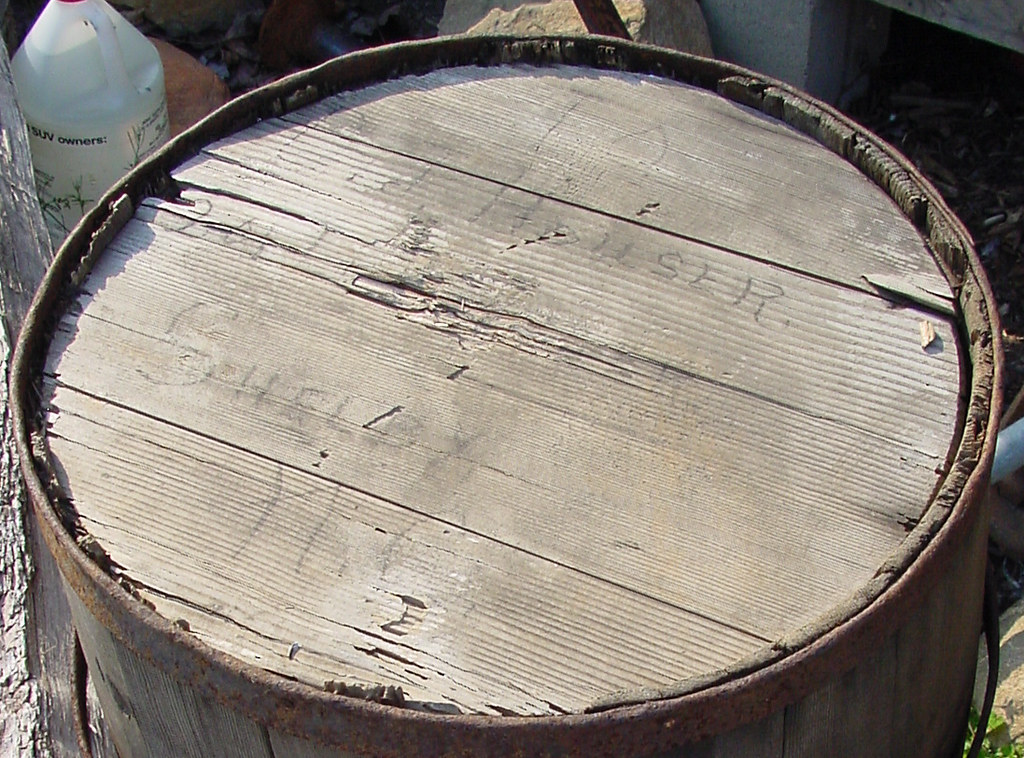The image depicts the top of a well-worn, light-colored wooden cask or whiskey barrel, featuring a rusted metal rim. The surface of the wood is faded to a grayish tone and is chipped, torn, and broken in several places. Inscribed on the top are the partially legible letters "H-O-U-S-E-R" and "S-H-E-L-B," seemingly reading "to Hauser from Shelby" in a light black marker. To the left of the cask, there's a plastic bottle with the label "SUV owners." In the background, towards the top-left, you can spot part of a rock and some dirt, while the upper-right side shows a more expansive dirt area. The scene gives the impression that the barrel might have been used as a drum or something of similar function, and it rests in a somewhat natural setting amidst a tree and rock.